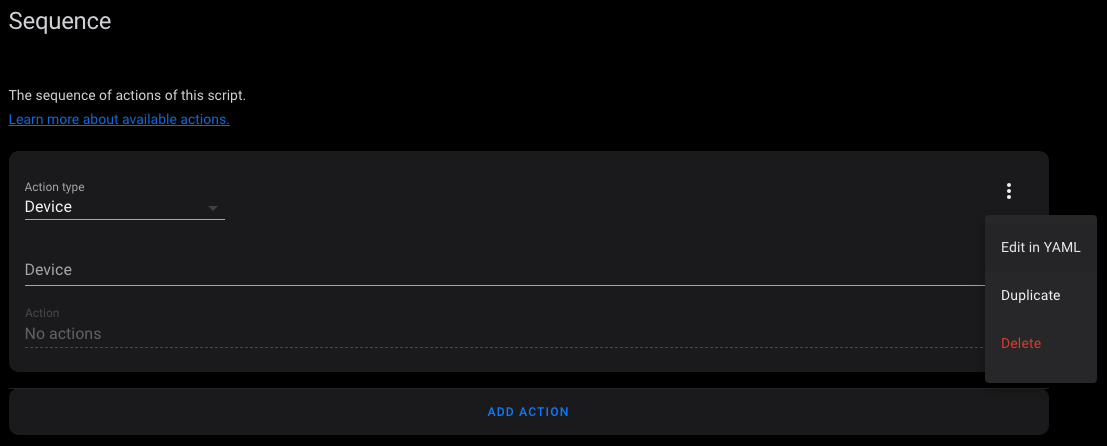**Caption:**

The screenshot captures the action sequence editor within a scripting interface, displayed in dark mode. At the core of the screen, a sequence of actions is being configured. The action type selected is "device," indicating that the subsequent steps are focused on device-related actions. On the action settings, a hamburger menu on the right provides options to edit the action in YAML, duplicate it, or delete it. Below the current action settings, a blue-text link allows users to add multiple actions to the sequence, facilitating comprehensive script customization. The interface's dark background contrasts with light text, offering a visually appealing and easy-to-read display.